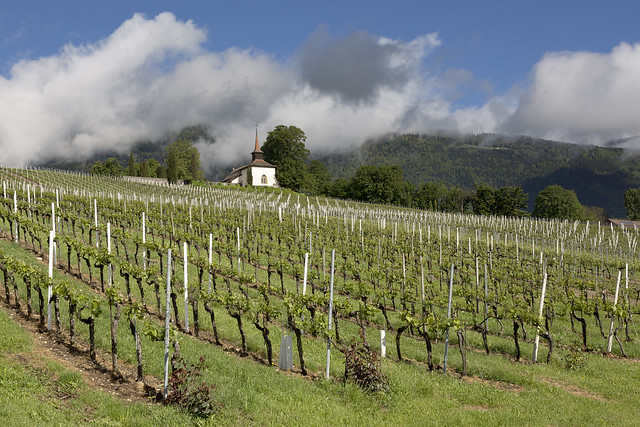The image depicts a newly planted wine vineyard stretching in neat, straight rows across the foreground. The crops are still in their early stages of growth, showing mostly roots and a few leaves. White posts can be seen intermittently amongst the plants, likely to support their growth. In the distance, slightly elevated, stands a picturesque small white church featuring a distinctive brown steeple. Surrounding the church are lush, dark green trees, creating a frame for the rolling hills beyond. The sky above is a striking contrast, with a bright blue expanse partially overtaken by dramatic, immediate storm clouds. The scene is devoid of human presence, highlighting the serene and pastoral beauty of what could plausibly be a vineyard in Italy, California, or Spain.